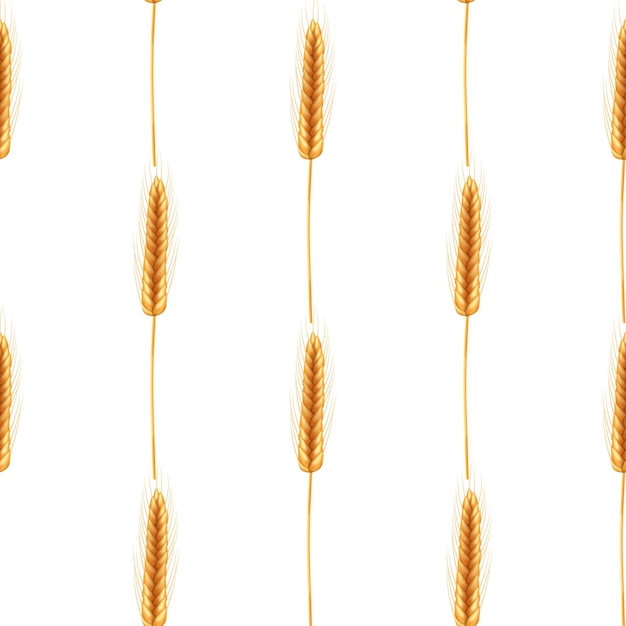This image features a detailed, artistically rendered depiction of plants resembling cattails or wheat, set against a predominantly white background with subtle beige tonalities. Each plant consists of a slender, brown, stem-like structure topped with a long, thin, rectangular cone-shaped object, which is golden brown in color. The tops of these structures possess delicate, wispy, light brown hairs or filaments extending outward, lending an intricate texture to the depiction.

Arranged in a vertical sequence, there are five distinct rows, each row showing multiple instances of these plants. The outermost rows on the left and right edges of the image are slightly cut off, revealing only parts of the plants, giving the composition a flowing continuity across the page. The plants are illustrated with a notable glow effect, making the yellow highlights more prominent and adding a sense of depth and dimension. This arrangement produces a visual rhythm reminiscent of pieces of wheat or cattails meticulously placed in rows, creating a harmonious and serene aesthetic.